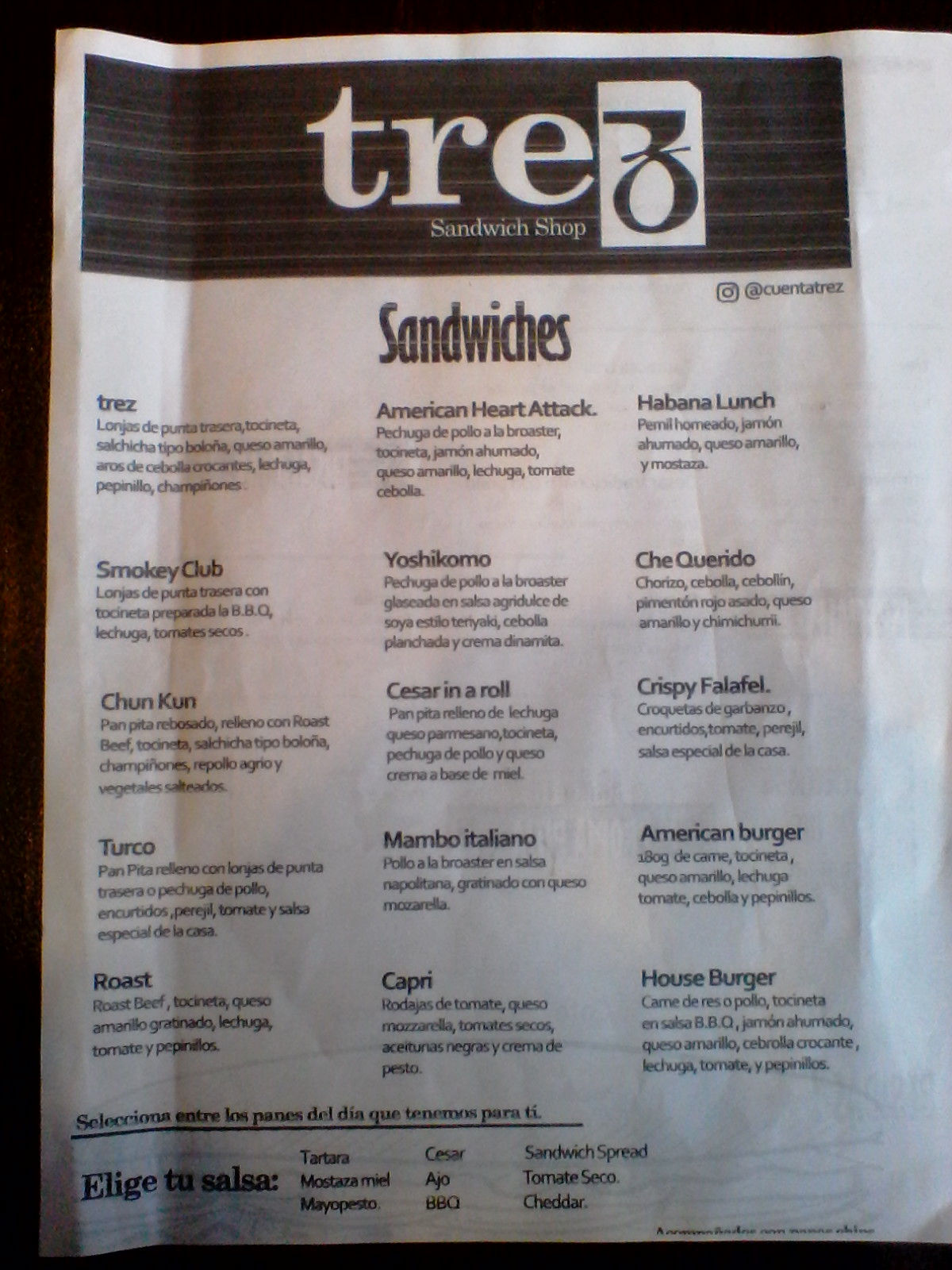A photograph captures a single-page sandwich menu printed on white paper, slightly creased vertically along the left side. The top of the menu features a dark-colored banner (possibly black, dark brown, or dark gray) with white text spelling "TRE." Within this banner, there is a distinctive brown numeral three inside a white rectangle. Below the banner, the text "sandwich shop" appears in small white letters.

The menu is titled "Sandwiches" and is organized into three columns, with approximately five sandwich options listed in each column. The sandwich names are a combination of English and Spanish, with the names in English and the detailed ingredients seemingly in Spanish. Here is a detailed list of the sandwich options provided:

**First Column:**
1. TREZ
2. Smokey Club
3. CHUN KUN (C-H-U-N, capital K-U-N)
4. Turco (T-U-R-C-O)
5. Panpita
6. Roast

**Middle Column:**
1. American Heart Attack
2. Yoshikomo (Y-O-S-H-I-K-O-M-O)
3. Mambo Italiano
4. Capri

**Third Column:**
1. Habano Lunch
2. Che Clarino
3. Crispy Falafel
4. American Burger
5. House Burger

At the bottom of the menu, under a partial line that creates a semi-boundary, it reads "Elige Tu Salsa," followed by additional items in Spanish.